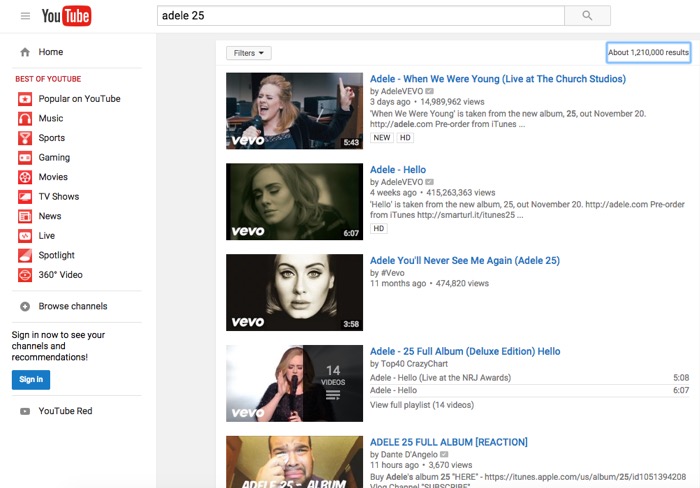**Caption:**

In this YouTube search for "Adele 25," the top results showcase various performances and reactions related to her new album "25," released on November 20th. The first video, "Adele - When We Were Young (Live at The Church Studios)," was uploaded three days ago by Vevo. It features an image of Adele singing with her pointer finger raised. The description highlights that "When We Were Young" is from the new album "25," available for pre-order on Adele.com and iTunes. 

The second video, "Adele - Hello," posted four weeks ago, also on Adele's album "25," shows a serene close-up image of Adele. This live performance at the NRJ Awards is listed as 6 minutes and 7 seconds long. 

The next result, "Adele - You'll Never See Me Again," posted one month ago by Vevo, details another song from the album with an image of Adele singing with her eyes closed and a hand to her ear. 

Additionally, a full playlist with 14 videos includes "Adele - Hello (Live at the NRJ Awards)" and a video titled "Adele 25 Full Album Deluxe Edition" by Top 40 Crazy Chart. 

One of the videos shows a man crying and dabbing a Kleenex to his eye, labeled "Adele 25 Full Album Reaction" uploaded 11 hours ago. The link to purchase or listen to the album on iTunes is provided (itunes.apple.com/us/album/25/id1051394208).